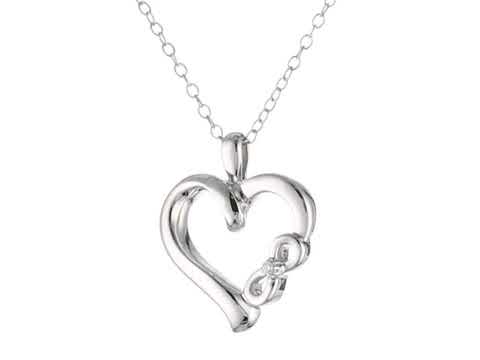The image features a silver necklace with a thin, round-link chain. The centerpiece is a heart-shaped pendant with a distinct design. The heart is open and has a thick frame, giving it a solid, substantial look. On the right side of the heart, an infinity symbol is integrated, symbolizing eternity or everlasting love. In the center of the infinity symbol, there is a small gemstone, which could be diamond or cubic zirconia. The pendant and chain are both crafted from silver, with no hints of gold or other colors. The background of the image is a clean, white slate, emphasizing the sleek and elegant design of the necklace. This close-up stock image aims to highlight the key features and craftsmanship of the jewelry piece.